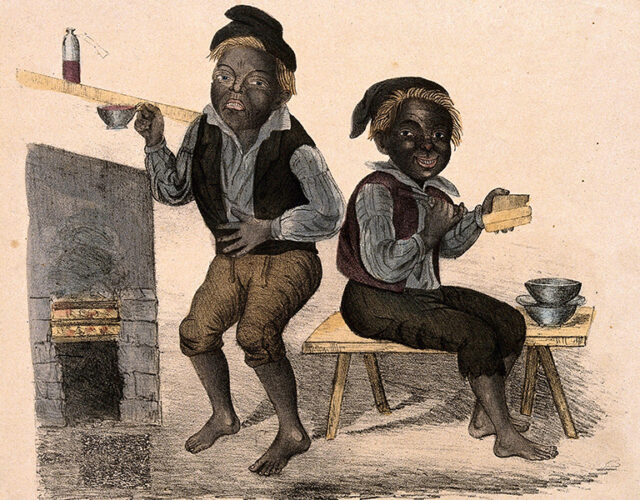The image depicts a room with creamy peach or pinkish walls and a small, black fireplace on the left side. In front of the fireplace stands a dark-skinned young boy with an agonized expression, holding his stomach with his left hand and a steel teacup in his right. He is adorned in a black vest, a light blue or gray long-sleeve shirt, and beige or brown shorts, with no shoes. Beside him is a wooden table or bench, on which sits another dark-skinned child wearing a similar black gnome-like hat, a black vest, and gray sleeves. This child has a cheerful smile, is looking directly at the viewer, and holds a piece of peach-colored bread-like food in one hand while the other rests on his heart. The room appears sparse, with a sense of vintage charm. Near the fireplace is a shelf bearing a bottle of liquid, completing the cozy yet humble scene.